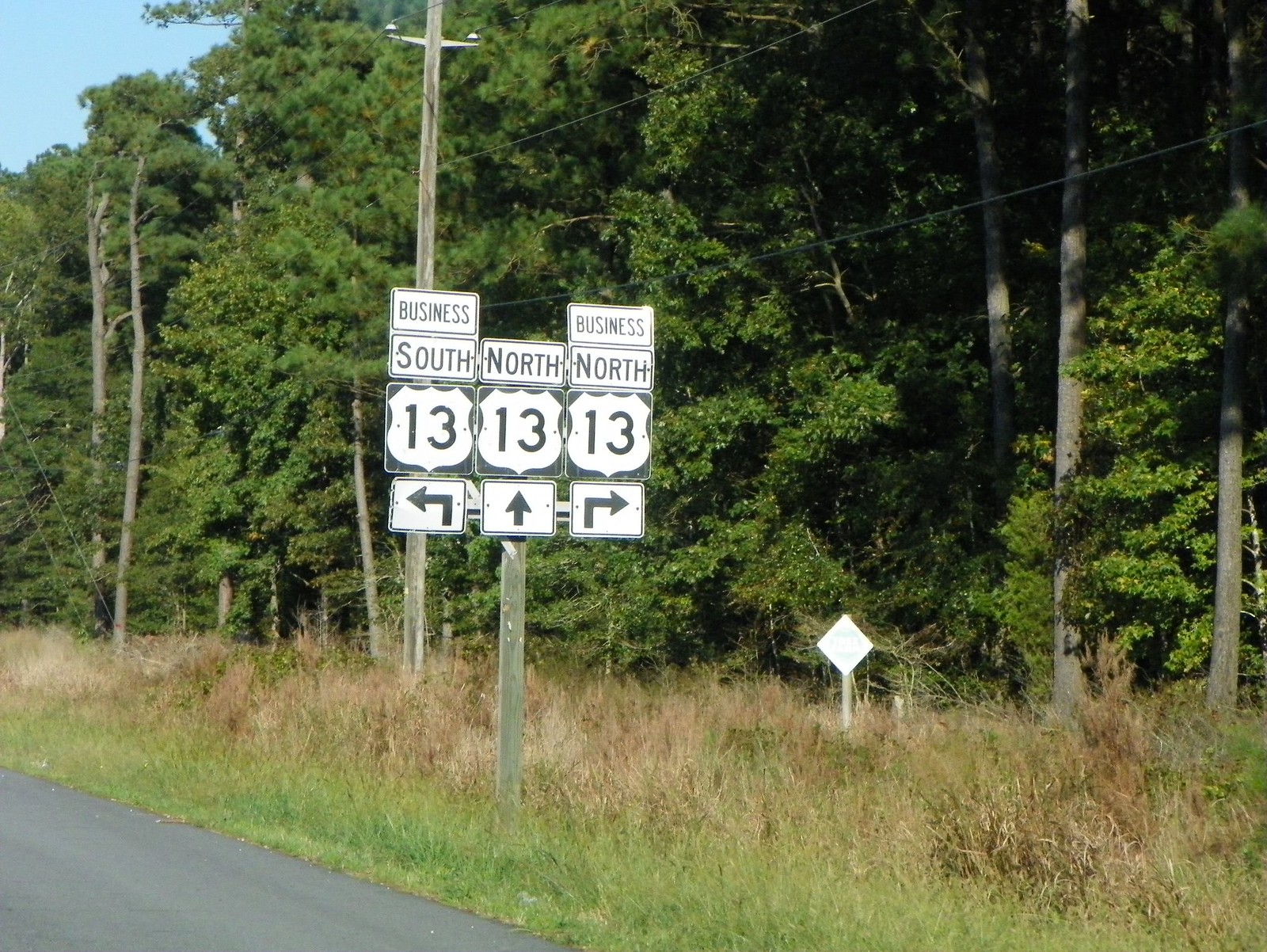The image captures a road sign indicative of U.S. Route 13, set against a perfectly clear blue sky in the upper left corner. The backdrop features a densely wooded area, with trees stretching across the entire image from left to right, and a strip of grass below. In the lower left corner, there is a small patch of blacktop pavement, confirming the location as the side of a road. The main road sign is mounted on a steel pole and comprises multiple directional indications: "Business South 13" with a left-pointing arrow, "North 13" with a straight-forward arrow, and "Business North 13" with a right-pointing arrow. Additionally, there is a diamond-shaped sign further back near the trees, though its message is unreadable. The scene is complemented by roadside elements such as grassy fields, weeds, and telephone poles with wires, contributing to the overall outdoor, rural setting.